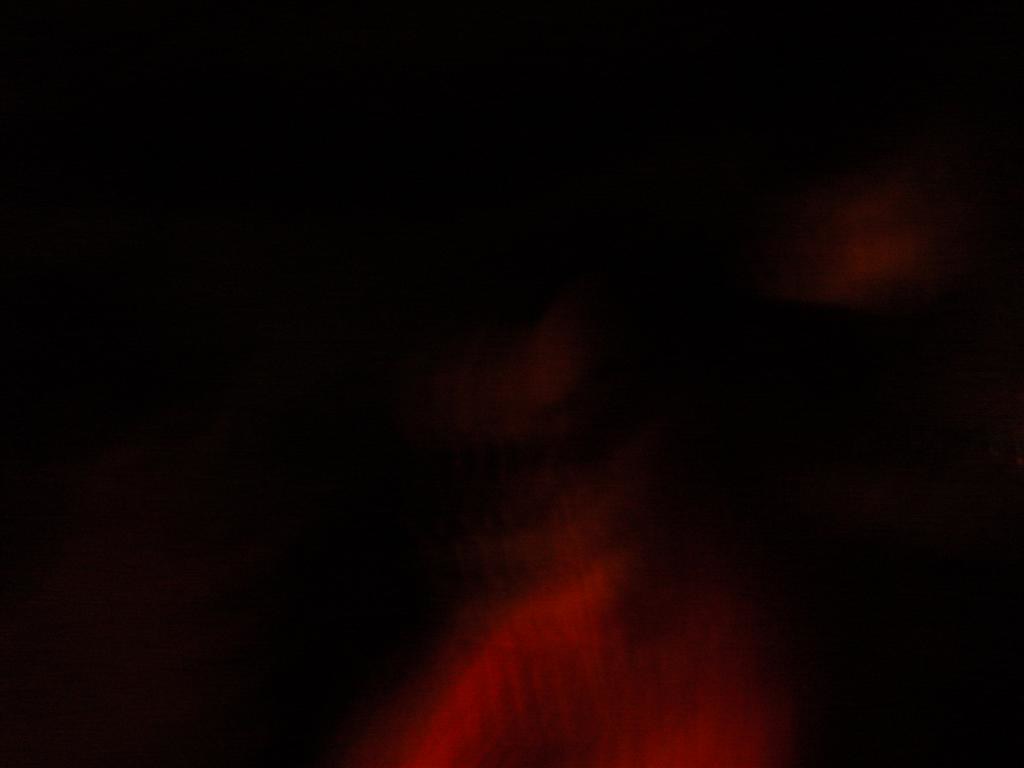The image is a low-resolution, blurry square, with the majority of its content being pitch black. Despite the poor quality and fuzziness, there are discernible patches of red at various points. Notably, at the bottom center, there is a darker shade of red, while a lighter red is situated above it at the mid-center. Additionally, another red patch is visible at the top right corner of the image.